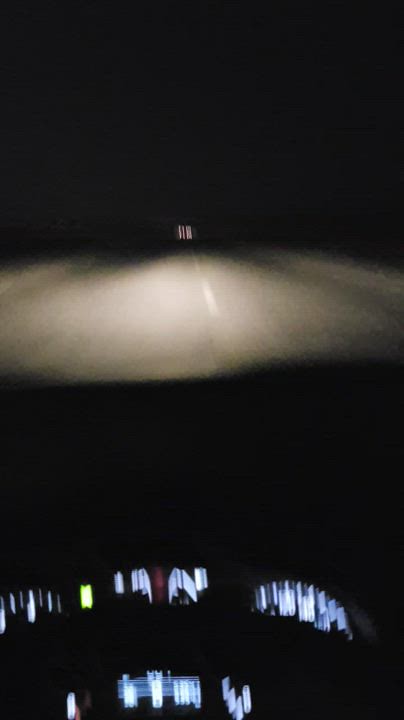The photograph captures the view from the driver's seat of a car at night, offering a dark, almost haunting ambiance. The top and bottom thirds of the image are enveloped in deep blackness, giving way to a slightly illuminated middle section where the headlights of the car cast light onto a two-lane road. Here, a solitary yellow dash line marks the center of the road, and faint curbs are discernible on either side.

The car's dashboard is visible in the lower portion of the image, its lights glowing amidst the darkness. Despite the blurriness, which suggests the car might be moving over a bumpy section of the road, certain details can be made out. To the left, the speedometer is lit up in white, though the numbers are unclear due to the motion blur. Nearby, there is a bright yellow illuminated rectangle, flanked on the right by another lit-up rectangle. Below and slightly to the left, a small area is lit, and beneath the steering wheel, another blue-lit rectangular space is visible.

In the distance, scattered lights—possibly from oncoming traffic or an electrical traffic sign—pierce through the inky darkness, adding a touch of intrigue to the mysterious and artistic nature of the photo. The blurred lines and indistinct shapes of the lights contribute to a sense of motion and disorientation, turning an ordinary night drive into an abstract visual experience.